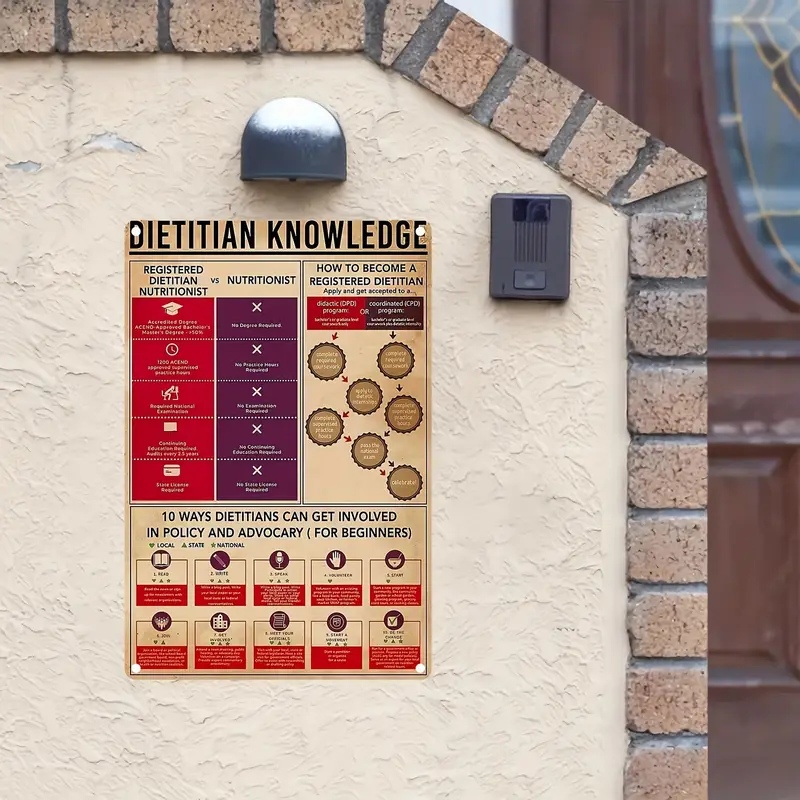This full-color outdoor photograph captures a beige stucco wall adorned with a large, square poster affixed by four thumbtacks, with a small tear revealing white drywall on the upper left side. The wall features a brown brick border separated by gray grout. Prominently displayed on the poster, in all caps and underlined in black, is the title "DIETITIAN KNOWLEDGE." The poster details the differences between a "Registered Dietitian Nutritionist" (highlighted in red) and a "Nutritionist" (highlighted in purple) in a side-by-side column format. It further explains "How to become a registered dietitian" and lists "Ten ways dietitians can get involved in policy and advocacy for beginners," outlined in two rows of five boxes each. To the right of the poster, there is a small, dark gray box that appears to be an alarm or speaker. In the background to the far right, a wooden entry door with an oval glass window and decorative brass elements is visible.